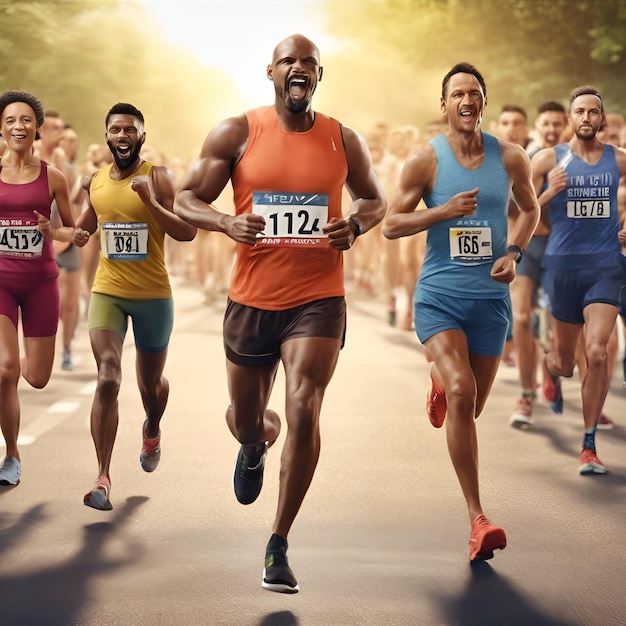The image depicts a surreal race scene that appears to have been generated by AI, featuring five runners in the foreground. The central figure is an African-American man wearing an orange shirt, numbered 112, and brown shorts. He has muscular legs, black shoes with white soles, and an incongruously wide-open mouth. Directly to his left is another African-American male in a yellow shirt, greenish pants, orange socks, and white shoes, although his features are distorted, making him appear disproportionately short. To the right of the central runner are two Caucasian males in blue shirts and shorts, both of whom have odd and unrealistic body proportions. 

To the far left of the image is an African-American woman in a red-pink attire, who similarly has an asymmetric and distorted face. The background is a blurred mixture of a sunlit landscape with trees and an indistinct crowd, contributing to the image's bizarre and dream-like quality. The scene is under a hazy light that gives it a triumphant yet eerie feel, with distorted digits and unrecognizable text on the runners' shirts. The runners themselves exhibit a strange array of anatomical anomalies, making the entire visual composition appear unsettling and otherworldly.